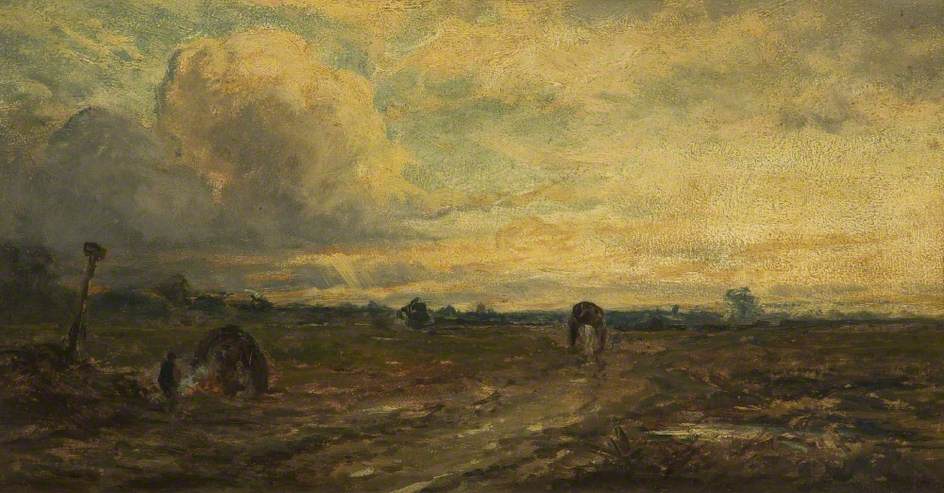This painting is a horizontally aligned rectangular canvas with a highly textured surface, giving a sense of roughness and age. Dominating the upper portion of the scene is a mostly overcast sky tinted in a mixture of grays, browns, and whites, with a distinctively large, fluffy cloud on the left transitioning into elongated, stretched clouds as they move right. The middle part of the painting transitions from sky to a barren landscape characterized by flat areas and subtle hills, rendered in subdued browns and yellows. 

In the foreground lies a desolate expanse, possibly representing a desert or worn farmland. The ground features rocky patches and sparse greenish areas, suggesting an eroded and weathered terrain. Among the indistinct shapes are hints of possible decay, such as crumbled structures. Notably, there is a potentially animal-like figure, maybe a cow, walking along the land. Close to the lower left side, a person identifiable by a small vest and hat appears to be standing near what could be a bale of hay or a tent. The figure might be tending to a small fire, hinted by a faint orange glow, surrounded by mostly abstract forms. Also sticking out of the ground is an ambiguous object, perhaps resembling a crooked sign or a tool. The overall image conveys a sense of age and decay, imbued with a melancholic atmosphere.